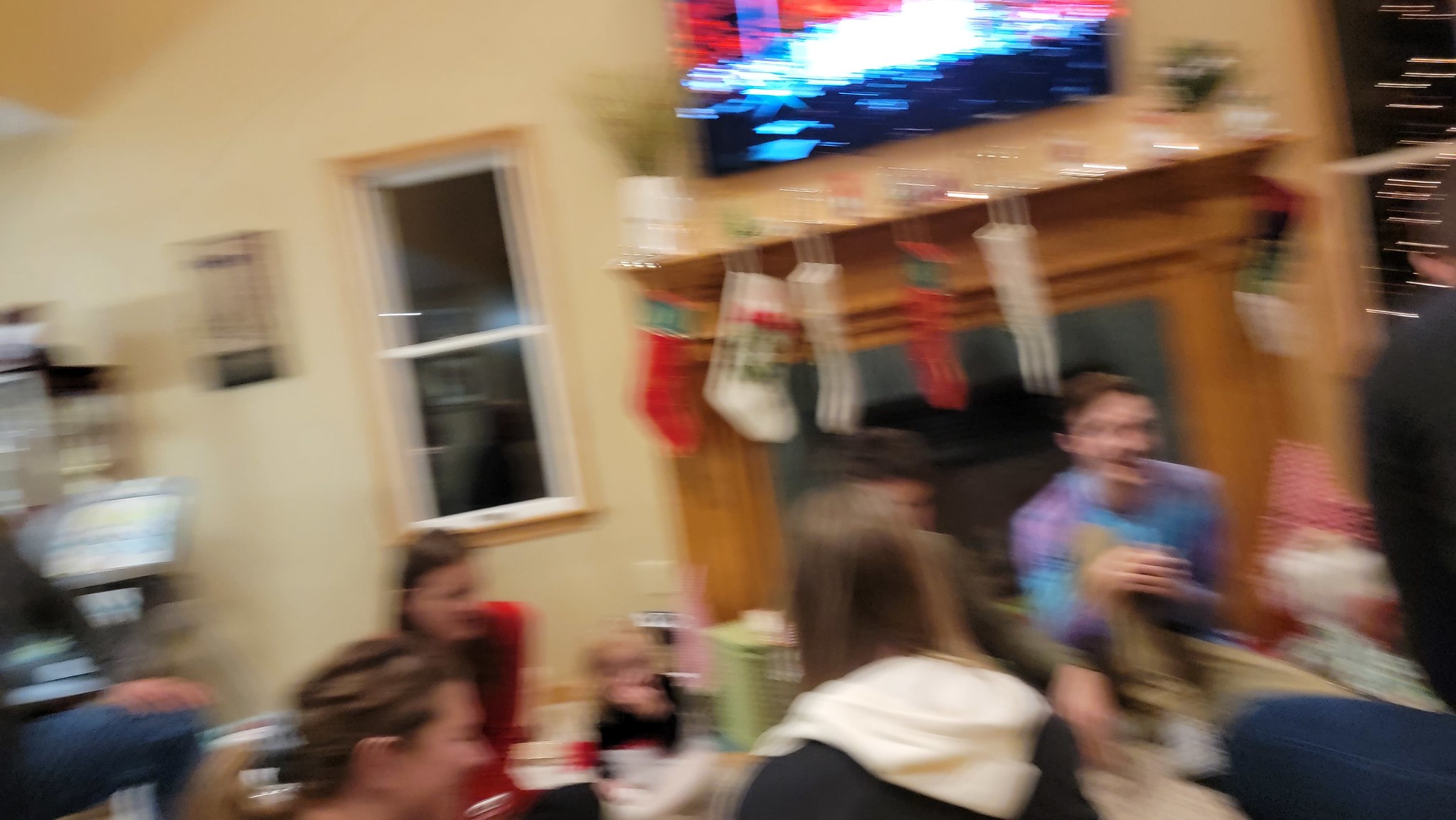In this completely blurred photograph, we glimpse the cozy interior of a home, possibly during a festive gathering. The scene appears to capture a moment at a party, where about five to six people are seated on the living room floor, perhaps engaged in conversation or a group activity. An additional figure, likely a child, is also visible, sitting on the floor in front of the fireplace. 

The individuals form a loose circle, facing each other amidst the warm, yellow-hued walls of the room. A window on the left side of the image allows some natural light to filter in. The focal point is the orange wood fireplace adorned with festive decorations; it features five or six Christmas stockings hanging from the mantle. These stockings are arranged in a sequence: red, white, white, red, white, and one on the far left that is red, green, and white. 

Above the mantle, partially cut off by the top edge of the photo, there appears to be a TV. Despite the heavy blur, which suggests the camera was moving when the picture was taken, the holiday spirit and intimate setting are tangible.